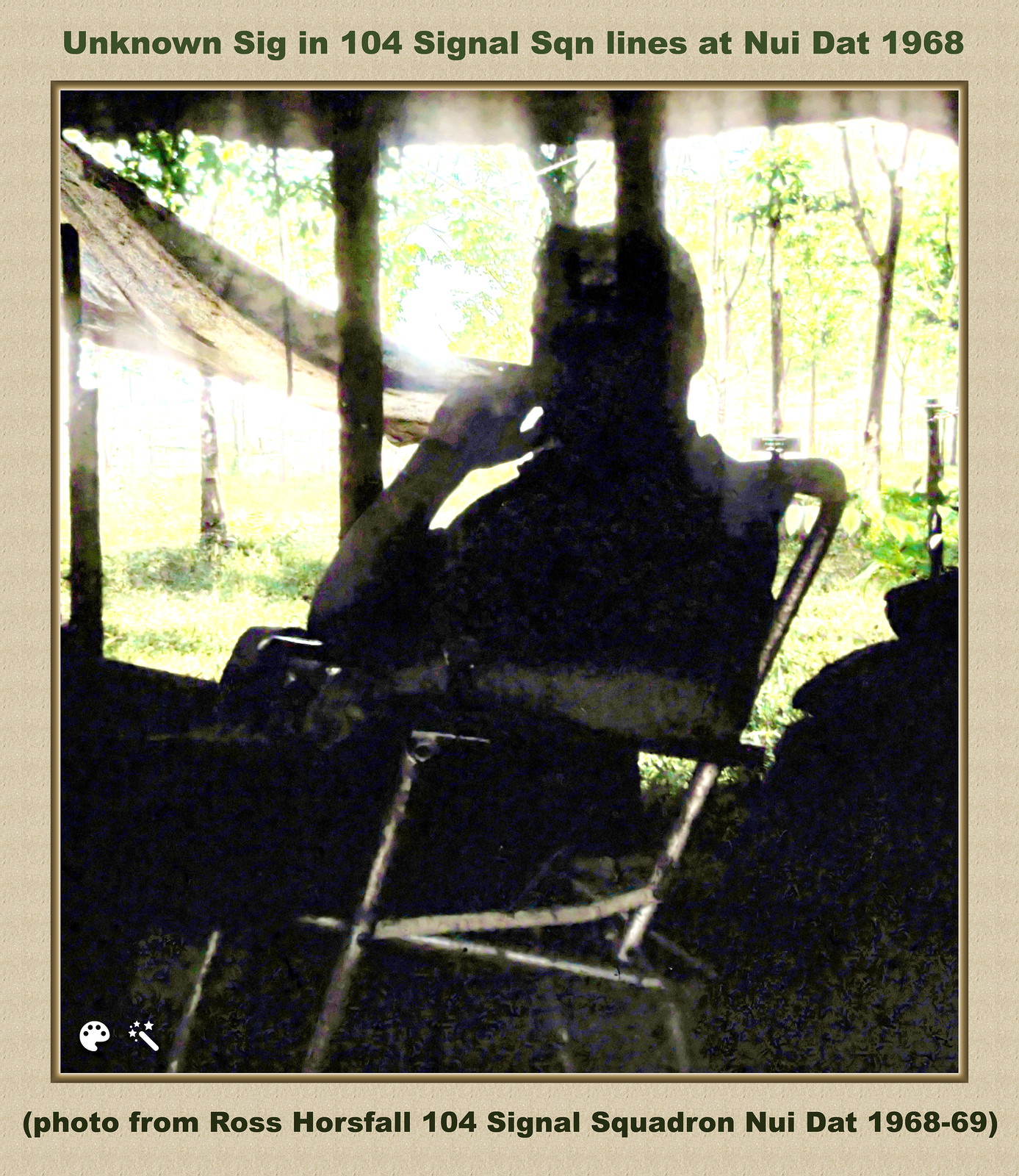This detailed photograph features a person seated in a metallic chair within a tent structure. The person is primarily obscured due to dark shadowing but is discernible with one hand resting on the chair’s armrest and the other hand on their face, appearing to be smoking. The tent opens to an outdoor area, revealing another tent and trees bathed in daylight. The image is framed by a light brown border, which contains text. The upper part of the border reads, "Unknown Sig in 104 Signal Sqn lines at Noydat, 1968," while the bottom states, "Photo from Ross Horsfall, 104 Signal Squadron, Noydat, 1968-69." The photograph includes a myriad of colors such as tan, green, brown, yellow, gray, black, and white. The scene likely depicts a moment from a military setting, possibly during the Vietnam War era, due to the references made to dates and signal squadrons. The man appears to be wearing a watch, and in the lower left corner, the image includes a paint pad with various colors, suggesting potential editing tools.